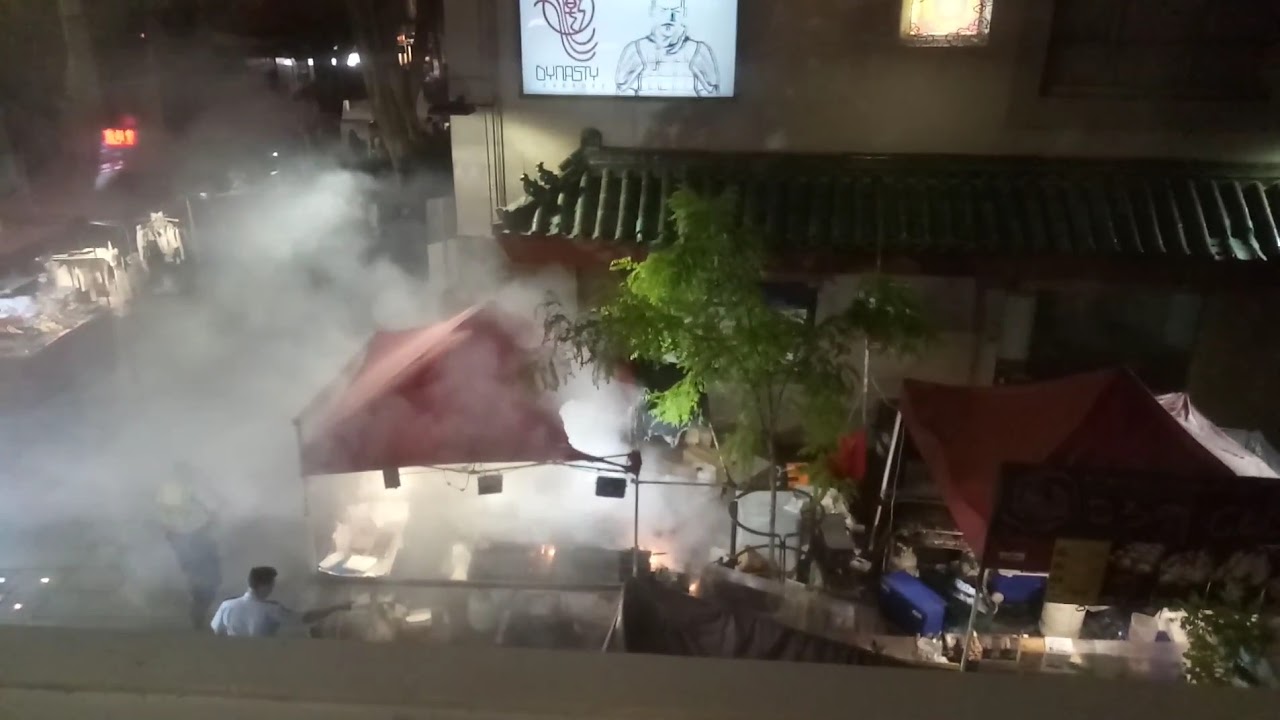The image captures a bustling nighttime scene at an Asian street bazaar, viewed from above. Central to the frame is a red food tent emitting thick, billowing smoke, possibly from grilling activities. The smoke obscures much of the scene and cascades towards the left and center of the image. On the left side of the frame, there are a few people walking and two men visible at the bottom left; one is reaching out while the other is shrouded in smoke, appearing as a silhouette.

Adjacent to the smoky tent, a small tree with green leaves and a couple of branches jut out, providing a hint of natural greenery amidst the urban setup. To the right of the smoky tent is another red tent without any smoke; the tent features a sign in shadows, likely displaying the menu.

In the background, the architectural style of the buildings hints at Asian influences, with notable features like green ceramic or stone tiles on the roof and cream-colored walls. Prominently displayed on one of these buildings is a white sign with the word "Dynasty" and a samurai-like figure. The scene conveys a lively yet slightly chaotic atmosphere typical of a street food market, enriched by the cultural elements and the nighttime setting.